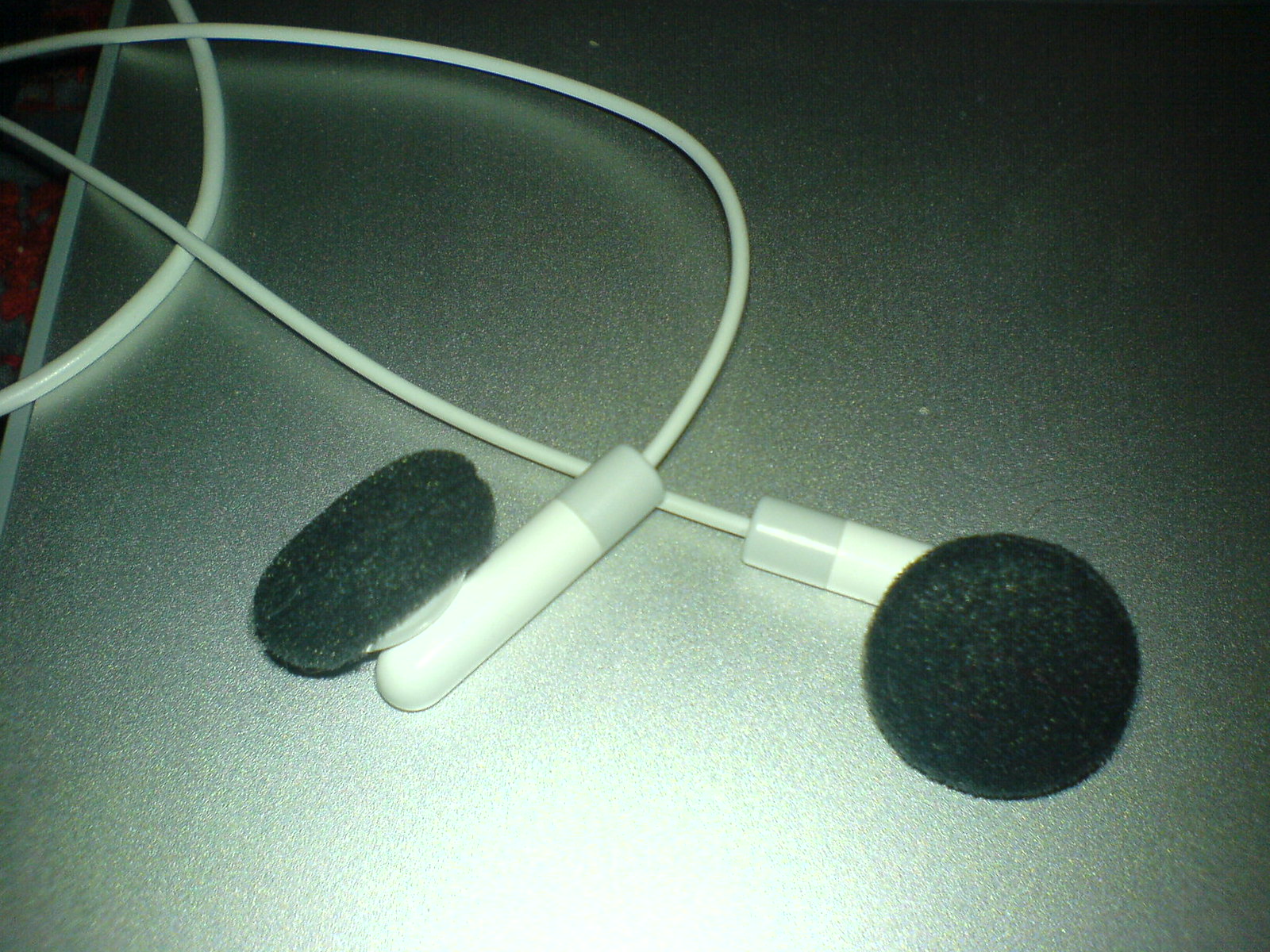In this black and white image, a pair of basic earphones is prominently displayed, contrasted against a metallic, grayish background that reflects light, adding a slight sheen to the scene. The layout of the earphones is meticulously detailed; they rest in the center of the image, with thin white wires emerging from either side. These cables loop and extend towards the upper left corner of the frame and towards the upper part, respectively.

The earphones are composed of white, pill-shaped capsules connected to cushioned, black circular earpieces made from a soft, fuzzy material. One of the earpieces is oriented straight towards the viewer, clearly showcasing its circular shape, while the other lies on its side, partially obscured by the first. The white wires blend seamlessly with the neutral-toned background, emphasizing the close-up and seemingly enlarged view of the earphones, making them the central focus of this otherwise minimalist composition.